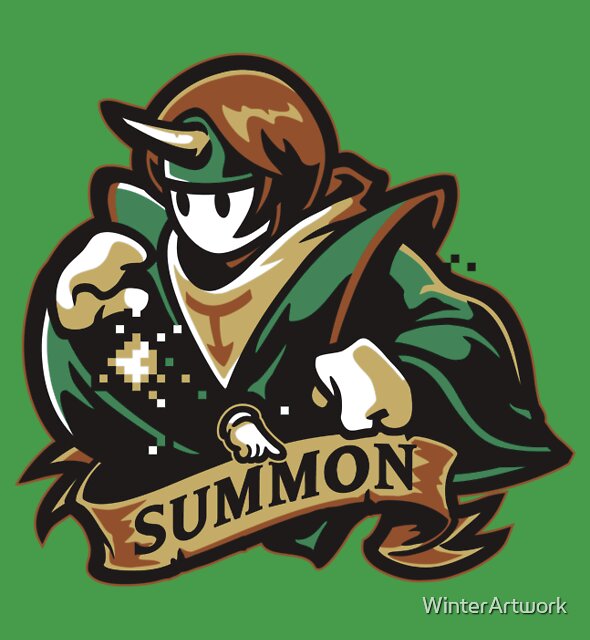The image features a vertically-oriented, slightly rectangular logo or illustration with a solid green background. At the center is a cartoon character dressed in a green robe over a brown sweater, complete with white sleeves and hands. Atop the character's head is a distinctive brown helmet with a white horn protruding forward, possibly complementing a green helmet beneath. The character holds a prominently displayed brown banner with the word "SUMMON" written in striking black letters. The entire image is heavily stylized with bold outlines and a color palette that includes green, brown, black, tan, and white. In the lower right-hand corner, small text reads "WINTER ARTWORK," possibly indicating a watermark or credit for the artwork, which might be intended for a show, game, or company logo. The character also has an additional shiny detail on their coat, positioned on the right side of the image.